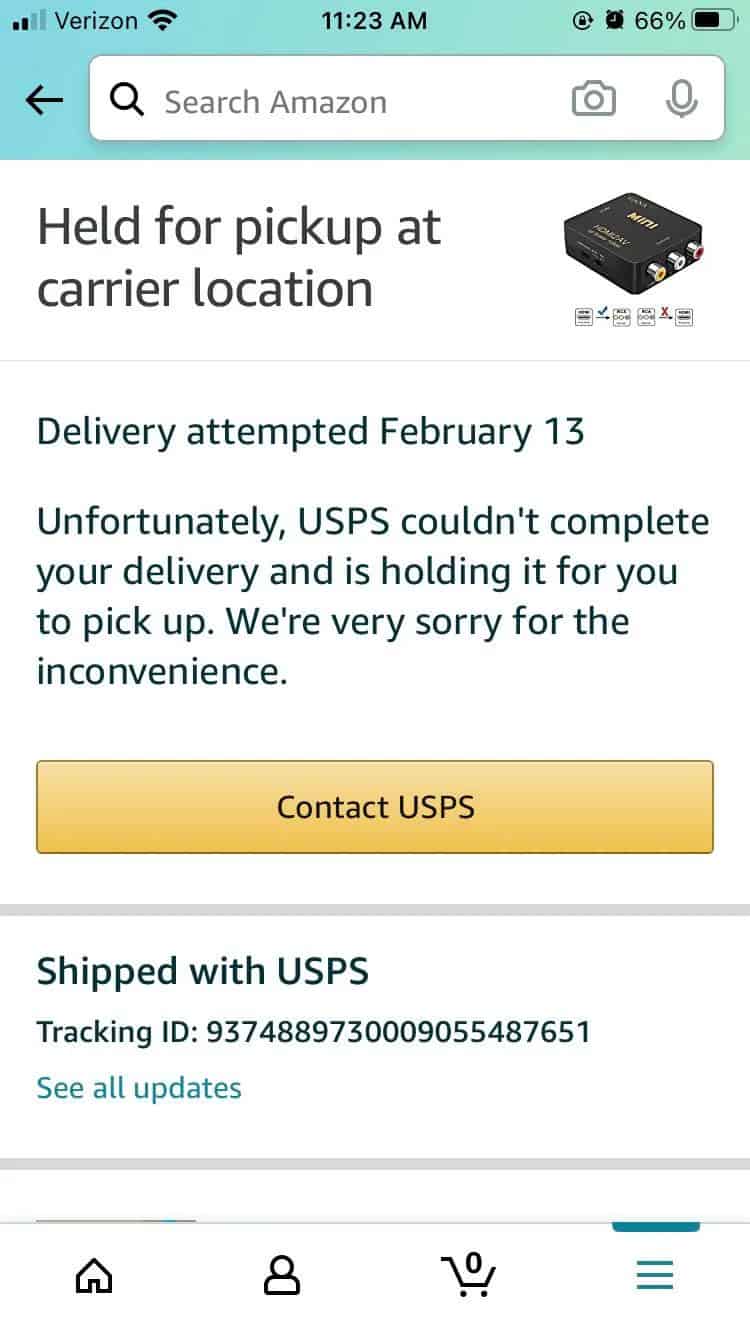A screenshot of the Amazon mobile app reveals a detailed delivery update. Prominently displayed at the top, the message "Held for pickup at carrier location" appears in large, bold, black letters. To the right of this message is a thumbnail image of the item in question. Directly below, written in bold green text, it states, "Delivery attempted February 13th." Following this, the app provides an apology, explaining that the delivery could not be completed but the package is being held for pickup.

Beneath this message, a large orange bar invites the user to "Contact USPS." Scrolling further down, the shipping details are given, indicating the shipment method ("Shipped with USPS") and the tracking ID. Additionally, small blue text below the shipping information offers an option to "See all updates."

At the very bottom of the screenshot, the phone's navigation options are visible. The top part of the screen features a blue-green search bar labeled "Search amazon.com," accompanied by a camera icon and a microphone icon on the right side. To the left of the search bar, an arrow provides a way to return to the main Amazon screen.